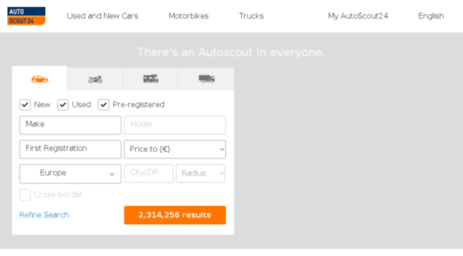This image is a low-quality screenshot of a webpage from AutoScout 24, slightly blurry but still legible. At the top left corner of the screenshot, there's the AutoScout 24 logo with "Auto" in blue and "Scout 24" in orange. Directly below the logo is a horizontal menu with the following items from left to right: "Used & New Cars," "Motorbikes," "Trucks," "My AutoScout 24," and "English."

The main content of the page is divided into a gray box and a white settings box within it. The gray box features a title in white text that reads, "There's an AutoScout in Everyone." Beneath this title, the white settings box offers four clickable tabs, each represented by different vehicle icons. The selected tab depicts a car and reveals specific search options.

Within the active tab, the first line contains three checkboxes, all marked with a check: "New," "Used," and "Pre-Registered." Below these checkboxes are input fields for refining the car search. The first field is for selecting the "Make" of the vehicle, followed by a grayed-out "Model" field. The next line includes "First Registration" and a dropdown menu for "Price To." Below these are two more fields: one for selecting "Europe" from a dropdown list, and two boxes for entering the "City/ZIP" and "Radius."

A gray checkbox labeled "Cross Border" appears under these fields but is currently unchecked. The final line of the settings box shows a clickable blue text for "Refine Search" and an orange box indicating the number of search results, which in this case reads "2,314,256."

In addition to the car tab, there are three other tabs for different vehicle types: a motorbike, a larger bus, and a semi-truck, though their settings are not displayed in the screenshot.

Overall, the image portrays a detailed search interface enabling users to filter their automotive searches with various parameters on the AutoScout 24 website.